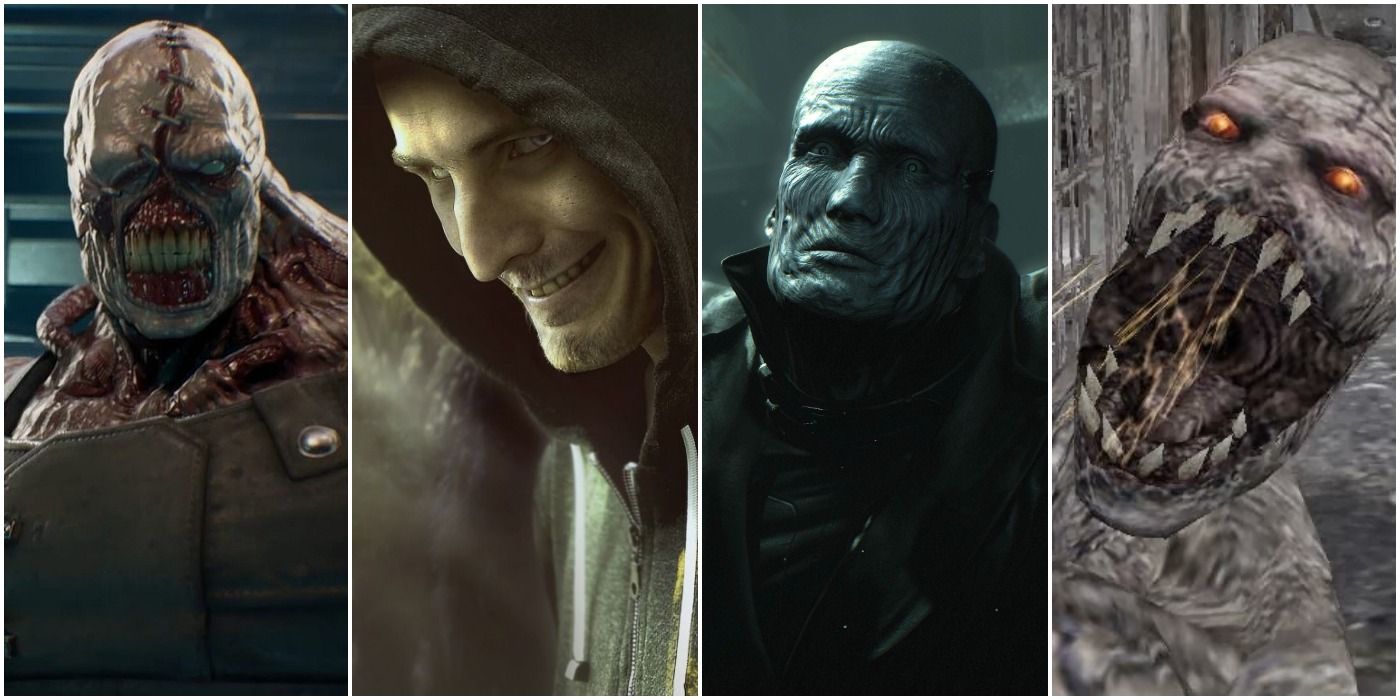The image features a series of four side-by-side high-definition screenshots displaying terrifying villains from the Resident Evil game series. Each villain's portrait is equally sized, tall, and narrow, creating a morbid gallery of ghastly faces.

From left to right:
1. The first villain is an incredibly gruesome, massive, and muscly creature whose head appears to be grotesquely stitched down the middle. The beast has no visible eyes; instead, its ravaged skin is pulled back to expose a cavernous mouth filled with pronounced teeth and red, bleeding gums.
2. The second villain is a sinister figure cloaked in a black hood, emanating an evil aura with his unsettlingly creepy smile and penetrating eyes.
3. Next is a hairless, stone-faced individual with a leathery, scarred complexion. His expression is vacant, looking slightly off to the side with a demeanor that contrasts the outright monstrosity of his predecessors.
4. The final image shows an eerily lifelike mummy-like creature with an enormous, gaping mouth. Its horrifyingly large fangs glisten with goo, and its red and yellow-orange eyes radiate a chilling malevolence.

Each character vividly embodies the eerie, dread-inducing atmosphere synonymous with the Resident Evil series.